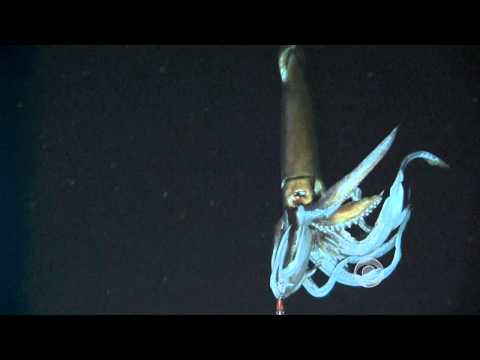Set against a grainy black background, an undersea photo captures a vertically oriented squid, with its tail up and head and tentacles down. The squid, positioned slightly off-center towards the right of the image, exudes an ethereal glow, particularly from its neon blue tentacles, suggesting photoluminescence. The body of the squid is illuminated, likely by the photographer's flash, revealing a dark olive-green hue, while its head is a lighter tan with green tinges. The head is narrow with visible eyes and transitions into long, splayed tentacles that shine with a neon blue glow, reminiscent of a vintage sign. A faint logo in the corner hints at a possible CBS video or image source, blending into the brassy but possibly silvery base of the creature, contributing to the mysterious allure of this deep-sea life encounter.